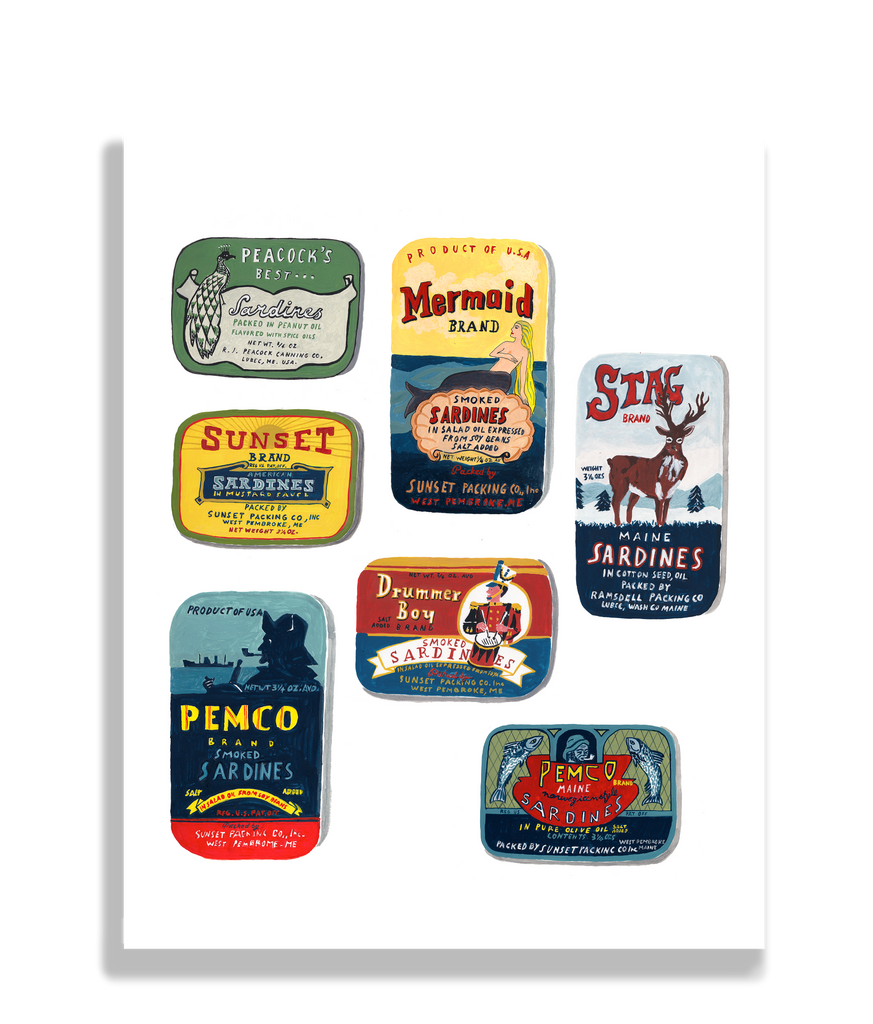This rectangular image, set against a plain white background with subtle gray shadowing along the left and bottom edges, showcases a collection of vintage sardine tins, each uniquely designed. 

Starting from the top left, the first can features a green background with white text reading "Peacock's Best Sardines," alongside a peacock illustration. Directly below it is a bright yellow tin labeled "Sunset Brand Sardines" in bold red and blue letters. Continuing further down, in the bottom left corner, there's a dark blue tin from "Pemko Brand," depicting a blue marine scene and a fisherman, labeled "Smoked Sardines."

Moving to the top center, there's a tin with a yellow top and blue bottom, branded "Mermaid Brand Smoked Sardines," featuring an illustration of a mermaid. Directly below it, a red-colored "Drummer Boy Smoked Sardines" tin is adorned with an image resembling a Christmas drummer boy. 

On the right side of the image, there is a tall, vertically aligned "Stagg Brand" tin with a light gray-blue background, showcasing a buck and labeled "Maine Sardines in Cottonseed Oil." Finally, at the bottom right, a "Pemko Maine Sardines" tin displays two fish placed opposite each other, with the label highlighted in red and yellow.

Each tin's design and vivid colors not only highlight the various brand names but also evoke a nostalgic glimpse into historical sardine packaging.